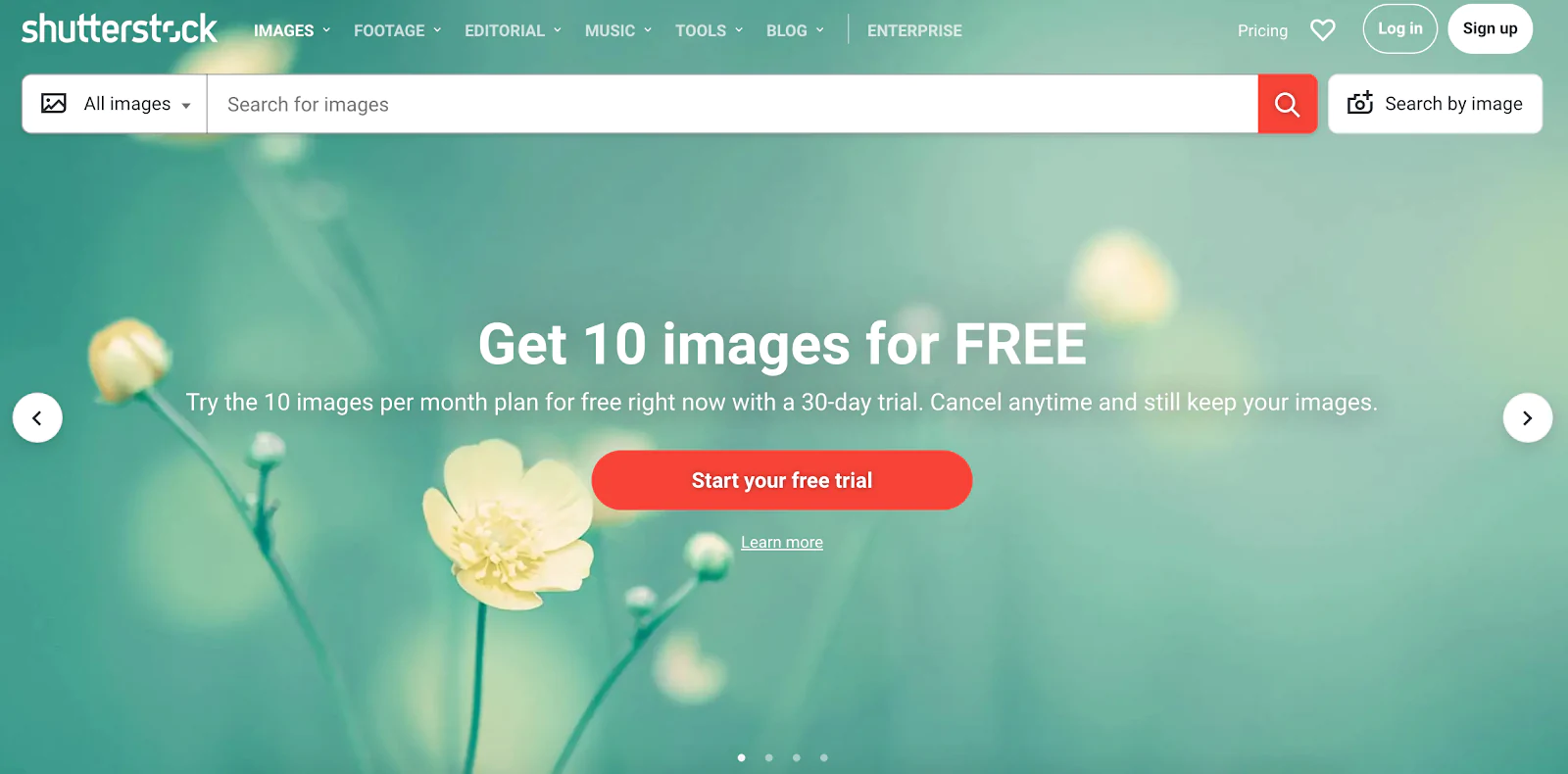This image, sourced from the website Shutterstock, displays a clean and user-friendly interface. At the top of the page, several drop-down menus are visible, including categories such as Images, Footage, Editorials, Music, Tools, Blog, and Enterprise. Below these menus lies a search bar with the placeholder text "Search for images," accompanied by a distinct red magnifying glass icon. The header also features options for pricing information, a heart icon for favorites, and login or sign-up buttons. Users can search by images as well.

The background color of the website is a soothing light greenish-blue, with a soft-focus image of yellow buttercup flowers taking center stage. The flowers are the focal point of the image, with the camera zoomed in on a few delicate buds, while the background remains artfully blurred to draw attention to the foreground elements.

Prominently displayed in the middle of the screen is an enticing offer: "Get ten images for FREE," with the word "FREE" in uppercase white letters. Below this, in smaller white text, the proposal clarifies: "Try the ten images per month plan for free right now with a 30-day trial. Cancel any time and still keep your images." A striking red button invites users to "Start your free trial," further enhancing the call to action.